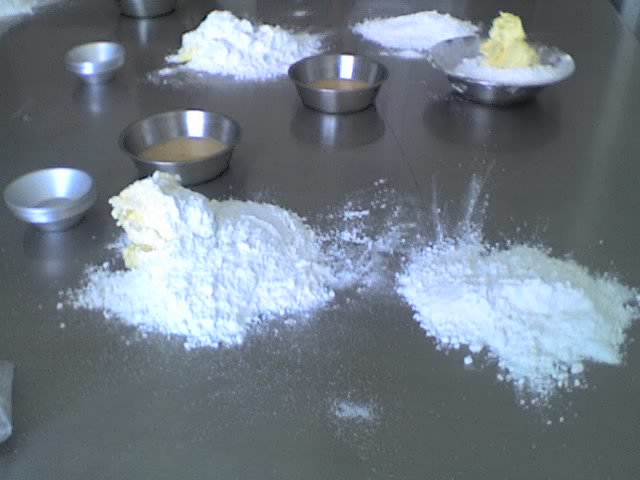The photograph captures an untidy culinary scene on a shiny metallic tabletop, reflecting several scattered metal bowls of varying sizes. Prominently, there are three main piles of a flour-like white powder spread across the table. Among these, four key bowls span the middle ground: the two on the left are small and empty, while the two in the center are medium-sized and contain a yellowish-brown liquid, possibly melted frosting or chocolate. The largest bowl on the right holds a mound of the white powder with a large, ambiguous yellow object on top, which could be a stick of butter or a scoop of ice cream. A hint of another pile of the white powder is visible in the upper left corner but is partly clipped by the photograph's frame. No people are present, and the setup does not appear to involve active cooking.